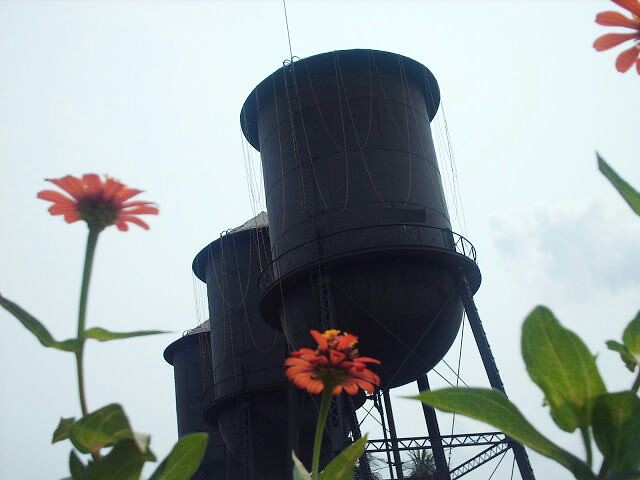In this photograph, we see three large black water towers positioned adjacent to one another, elevated on pedestals with legs. Each tower is interconnected with various cables or electric wires running off the sides and the top, contributing to their intricate appearance. The foreground features vibrant flowering plants, adding a striking contrast to the industrial structures. On the bottom left, there's a pinkish lily with delicate petals, while to its right, a bright orangish-yellow flower stands out, showcasing radiant orange petals. Surrounding these flowers is lush green vegetation, indicating a healthy, well-watered environment. The sky above the water towers appears clear, with a slight overcast, subtly softening the scene. The overall composition highlights the juxtaposition of the mechanical and natural elements, with the three black water towers prominently centered amidst a vivid display of flowering plants.